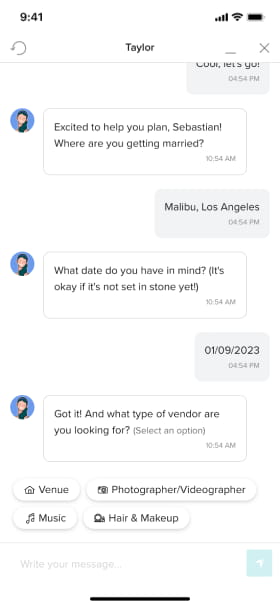A detailed screenshot of a smartphone interface is shown against an all-white background. At the very top, the device's status bar displays the time as 9:41, though it is unclear whether it's a.m. or p.m., with a strong implication that it's a.m. due to the bright background. The status bar also shows full signal strength with four bars and a fully charged battery.

Just below this, a refresh button sits centrally aligned. Beneath the refresh button, the name "Taylor" is clearly visible, flanked by icons for minimizing or exiting the screen. Further down, a messaging thread is presented, likely among users planning a wedding.

The conversation begins with a message: "Cool, let's go." Following this, a response from a user represented by an avatar reads, "Excited to help you plan. Sebastian, where are you getting married?" The reply is "Malibu, Los Angeles," to which another message asks, "What date do you have in mind? It's okay if it's not set in stone yet." This is followed by the date, "January 9th, 2023." Next, the conversation progresses with, "Got it. And what type of vendor are you looking for?" 

An option labeled "Select" is provided, allowing the user to choose from various vendor categories. A series of clickable buttons is displayed, including options for "Venue," "Photographer/Videographer," "Music," and "Hair and Makeup," offering the user multiple choices to aid in wedding planning, possibly through the assistance of an AI.